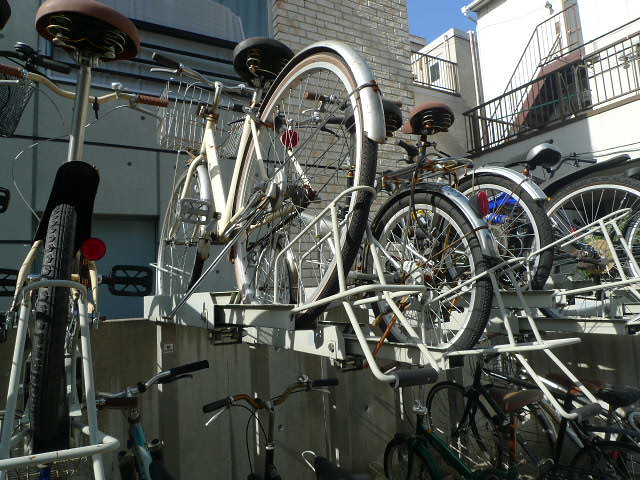In this sunny outdoor photograph, there is a two-tiered bike rack system located in front of a building complex. The complex includes a white brick building on the left and a white smooth-surfaced building with a staircase and railing on the right. The bike rack, designed for commuter bikes, features several metal struts that elevate some of the bikes, creating an organized yet densely packed appearance. The bikes themselves are predominantly white and gray, equipped with comfortable seats, medium-width tires, metal-framed baskets, and fenders over both the front and rear tires. Sunbeams and shadows play across the scene, highlighting the old-timey design of the bicycles, which evoke the feel of city bikes commonly used in places like Amsterdam.